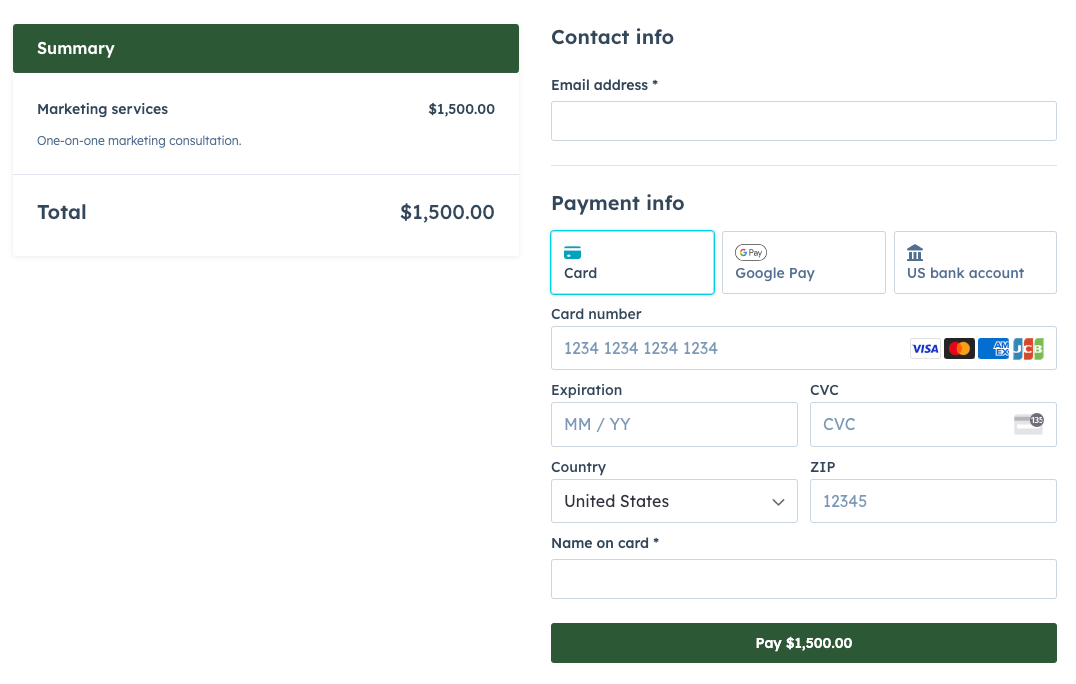This image depicts a billing and payment page with a predominantly white background. 

### Left Section:
- **Top Left Corner**: A black border with the word "Summary" in white text.
- **Below the Summary**: It reads "Marketing Services, $1,500.00" followed by "One-on-one marketing consultation."
- **Total Amount**: This section concludes with the text "Total $1,500.00" in black.

### Right Section:
- **Contact Info**: The heading "Contact Info, email address" is followed by an empty text box.
- **Payment Info**: The section starts with the heading "Payment Info."
  - **Payment Methods**: Three rectangular icons are presented:
    1. **Card Icon**: A rectangle with a blue border containing a card image and the word "Card."
    2. **Google Pay Icon**: A rectangle displaying the Google Pay logo.
    3. **U.S. Bank Account Icon**: A rectangle with a bank image, labeled "U.S. Bank Account."
  - **Card Information**: Several text boxes follow:
    - **Card Number**: Entered as "1234 1234 1234 1234."
    - **Expiration**: Displayed as "MM/YY."
    - **CBC**: Followed by "CBC" in the respective box.
    - **Country**: "United States" selected in the dropdown menu.
    - **ZIP Code**: Displayed as "12345."
    - **Name on Card**: An empty text box for the cardholder’s name.
- **Pay Button**: At the bottom, there is a dark green rectangular button with "Pay $1,500.00" centered in white text.

This detailed layout ensures clarity and helps users navigate the billing and payment process efficiently.